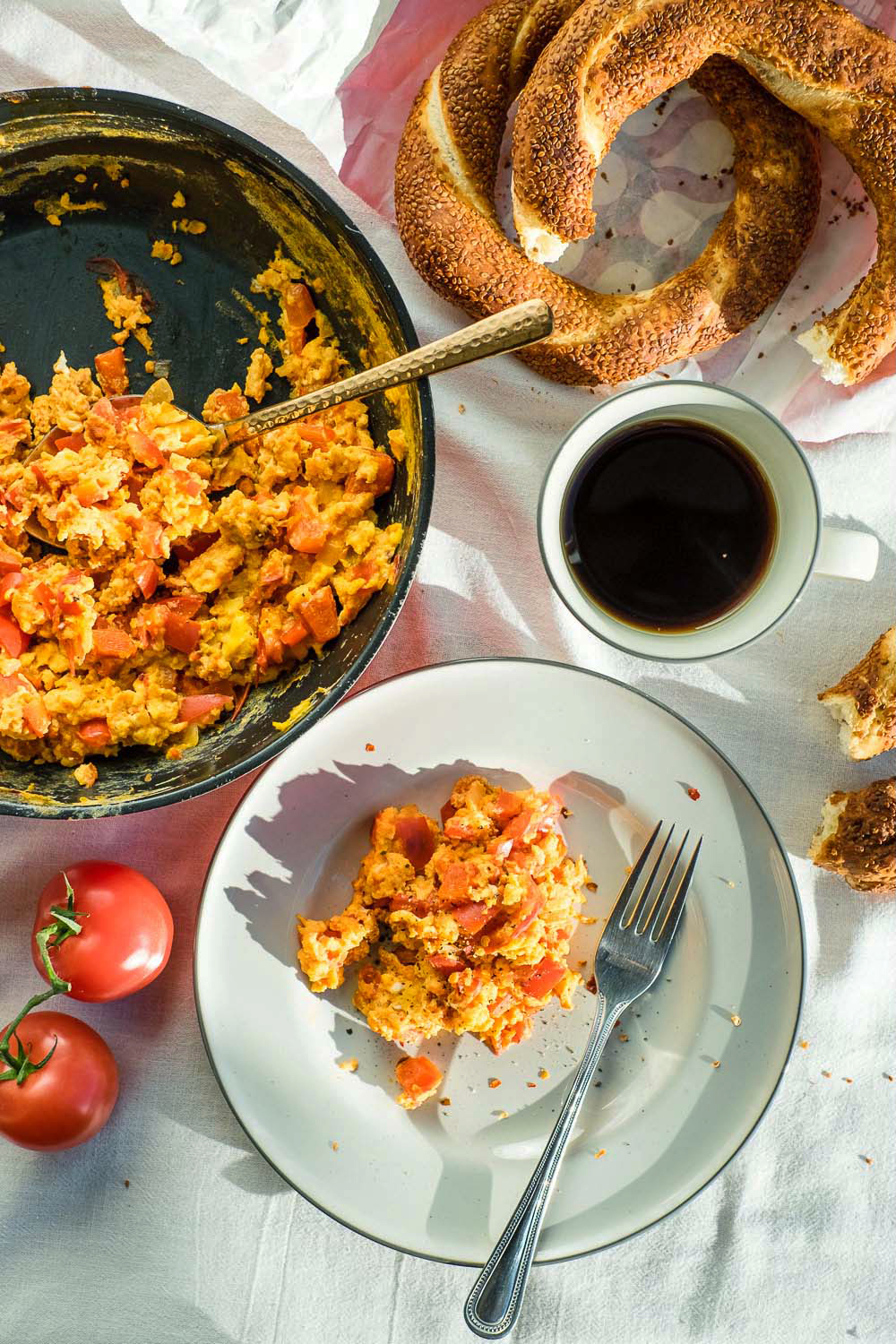The image is a meticulously arranged, top-down view of a breakfast spread on a white tablecloth, capturing the essence of a homemade recipe. Central to the composition is a large, black cast-iron skillet filled with a richly colored egg and tomato casserole, indicated by the bronze spoon peeking out. Adjacent to the skillet, two vine-ripened tomatoes add a fresh accent. To the right, a pristine white china cup with a black rim brims with steaming coffee. Above the cup, two ring-shaped bread pieces, adorned with sesame seeds, rest with one partially broken to reveal its fluffy interior. Below, a white plate with a black rim, paired with a silver fork, holds a neatly served portion of the casserole, mirroring the skillet's contents. The scene is bathed in warm sunlight, enhancing the inviting look of this hearty breakfast setup.